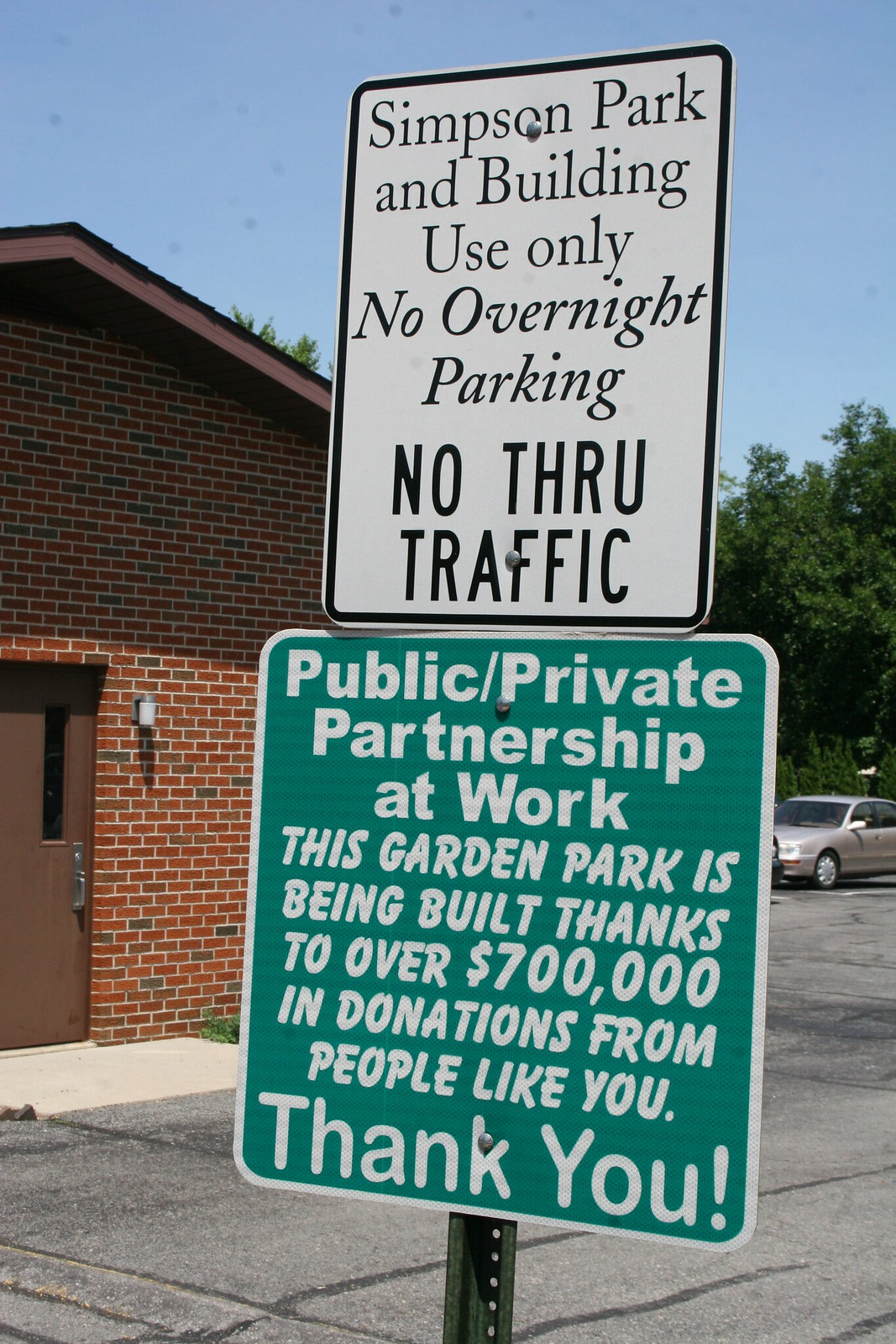The image is a daytime outdoor photograph featuring a parking sign mounted on a tall black metal pole. The scene is set in a parking lot with clear blue skies overhead. In the background, there is a large brick building with a brown wooden door and a light fixture beside it. The lot also contains parked cars and is surrounded by trees and greenery.

The parking sign consists of two parts. The top part of the sign is white with black text and a black border. It reads: "Simpson Park and building use only. No overnight parking. No through traffic." Notably, "No overnight parking" is italicized, and "No through traffic" is in bold. Below this, the second part of the sign is green with white text. It states: "Public/Private Partnership at Work. This garden park is being built thanks to over $700,000 in donations from people like you." At the bottom of the green sign, in larger white font, it says, "Thank you."

Overall, the photograph captures the essence of community involvement in the garden park project while enforcing parking regulations.